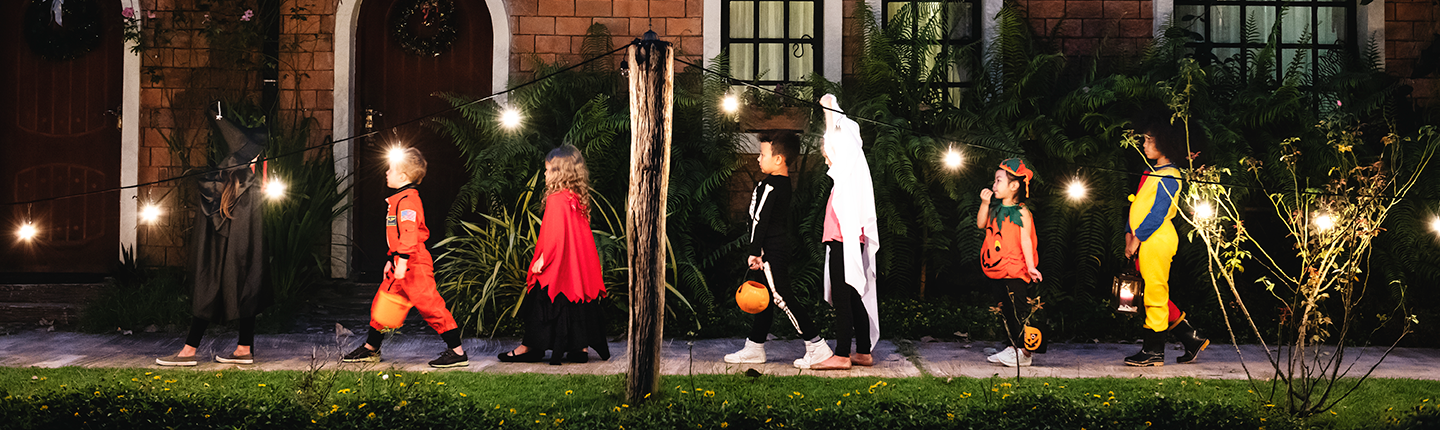In this horizontally elongated photograph, small children dressed in Halloween costumes walk along a narrow concrete pathway next to a brick-faced residential building. In the very foreground, a small strip of grass dotted with autumn-colored leaves stretches across the bottom edge of the image. The children, captured from their left side as they move from right to left, are bathed in the warm glow of string lights hung from a nearby wooden pole that faintly illuminates the nighttime scene. 

Leading the line is a child dressed as a witch, complete with a pointed hat and a flowing silk cape. Following her, a boy strides in an orange astronaut uniform, clutching an orange plastic bucket for collecting candy. Next is another girl in a witch costume, distinguishable by her red cape and black dress. Also visible is a child in a skeleton outfit, a black sweat ensemble adorned with white bone prints, and an Asian boy adorned in a pumpkin costume with a round body suit and hat. Finally, a little girl in a colorful clown outfit with yellow, red, and blue segments brings up the rear, adding to the festive parade of small, excited trick-or-treaters.